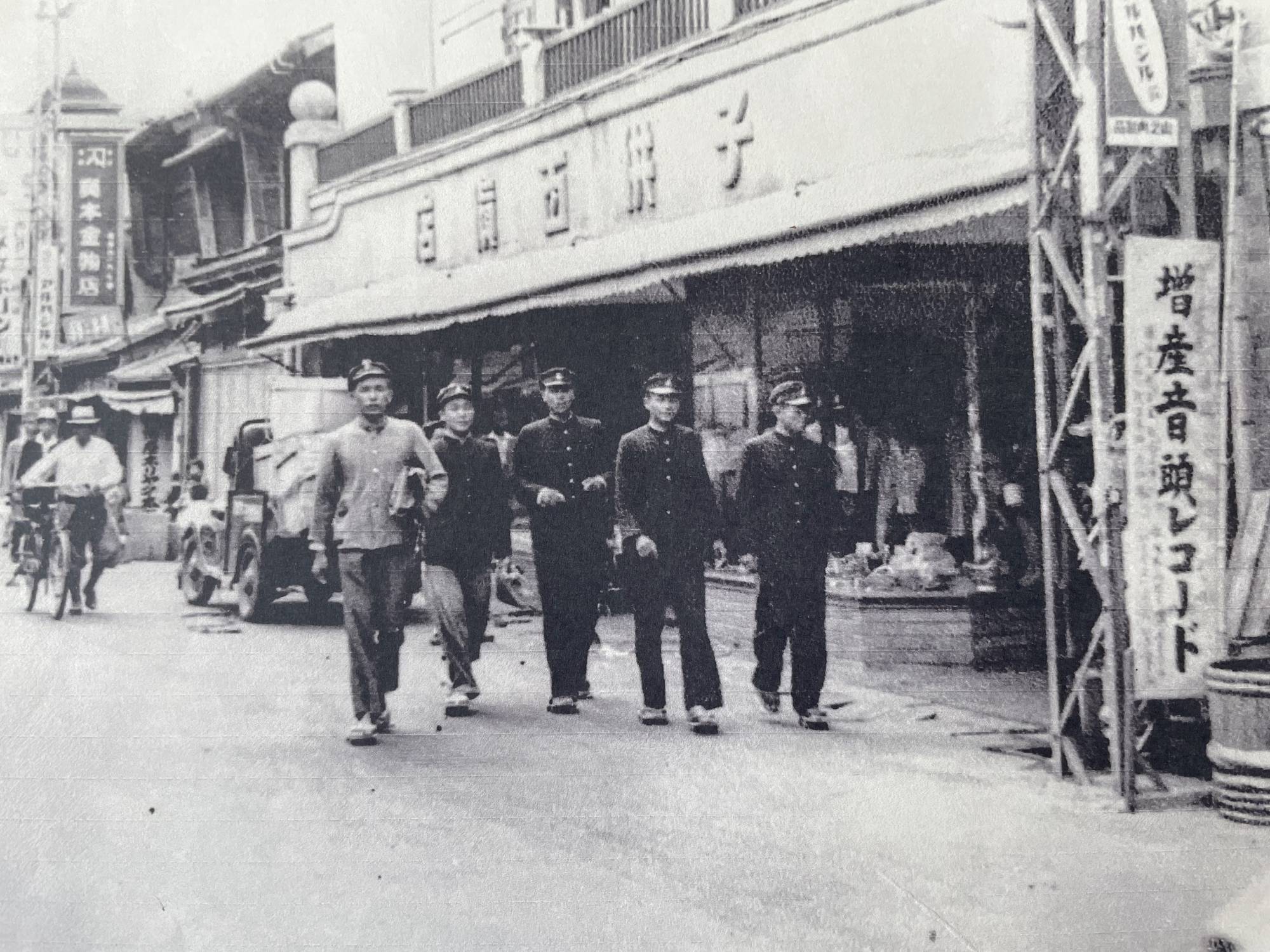This black and white photograph captures a historical street scene in an Asian city, likely Japanese or Chinese, as indicated by the intricate characters on the signs and buildings. Central to the image are five men dressed in formal attire, including official hats that resemble military or state uniforms, walking in a single file line toward the camera. All but one are clad entirely in black suits. The men, who may be officials or soldiers, are distinguishable by their hats and sandals. In the background, the street reveals additional activity: a truck loaded with crates is parked in front of a store window displaying clothing, and several individuals are seen walking or pushing their bicycles. The street itself appears moderately populated, reflecting a bustling yet orderly atmosphere reminiscent of mid-20th century urban life.